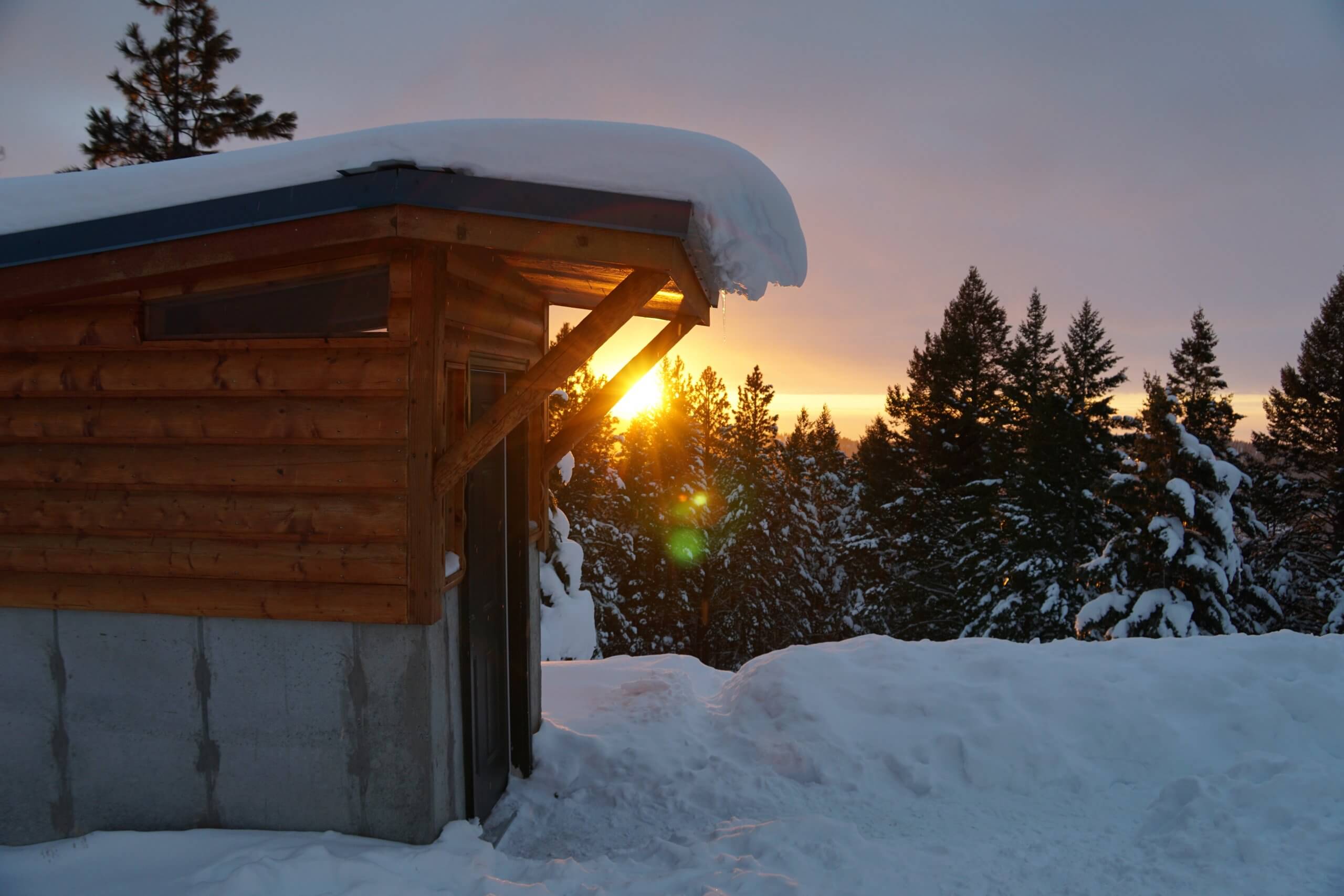This photograph captures a serene winter scene at either sunrise or sunset, featuring a small wooden shed situated in the foreground to the left. The shed has a concrete base and a horizontal log structure, crowned with a slanted wooden roof covered by about a foot of snow. Two angled wooden beams support the roof's metal eaves. A small trapezoidal window punctuates the top of the log wall, while a door faces the right side of the image. Snow piles up around the shed, and the ground shows signs of being recently dug out to allow access.

In the background, a dense forest of dark evergreen trees, heavily laden with snow, stretches across the scene. The tops of the trees reveal glimpses of their dark branches peeking through the snow. The sky overhead is a tapestry of colors, with blue clouds tinged in pink from the sun's light. The sun itself, a golden orb, sits just above the horizon, casting a warm yellow stripe of light and creating a lens flare with hues of orange, lime green, and dark green that radiate towards the center of the image. The entire photo is sharply focused, capturing every detail of this tranquil wintry landscape.